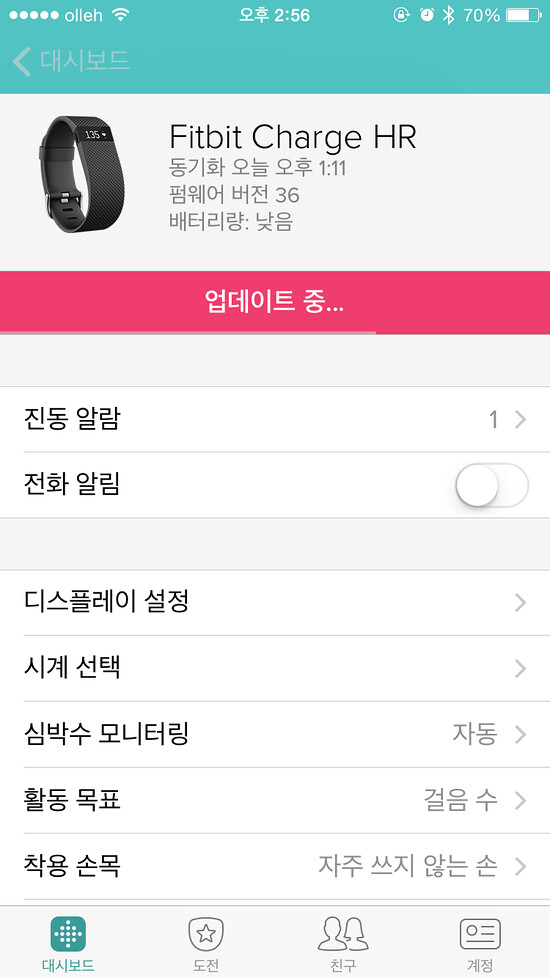The image is a screenshot from a smartphone likely using a retail app to buy a Fitbit Charge HR, displayed prominently in English among predominantly Korean text. On the top left of the screen is a black Fitbit Charge HR with a small digital face displaying a heart rate of 135, and to the right, the text "Fitbit Charge HR." The screen's upper section includes various status icons showing a 70% battery level, a Wi-Fi connection to the OLLEH network, Bluetooth turned on, an alarm set, and the time, 2:56. Below the product name, there are three rows of Korean text followed by a pink rectangular section also containing a Korean phrase. Further down, additional Korean text is arranged in several rows. At the bottom of the screen are four icons, including a green square on the left with a white diamond inside. The screen also features a blue button and possibly review-specific icons, indicating interactive elements typical of a shopping app interface. The overall color scheme includes shades of gray, white, tealish blue, and pink.